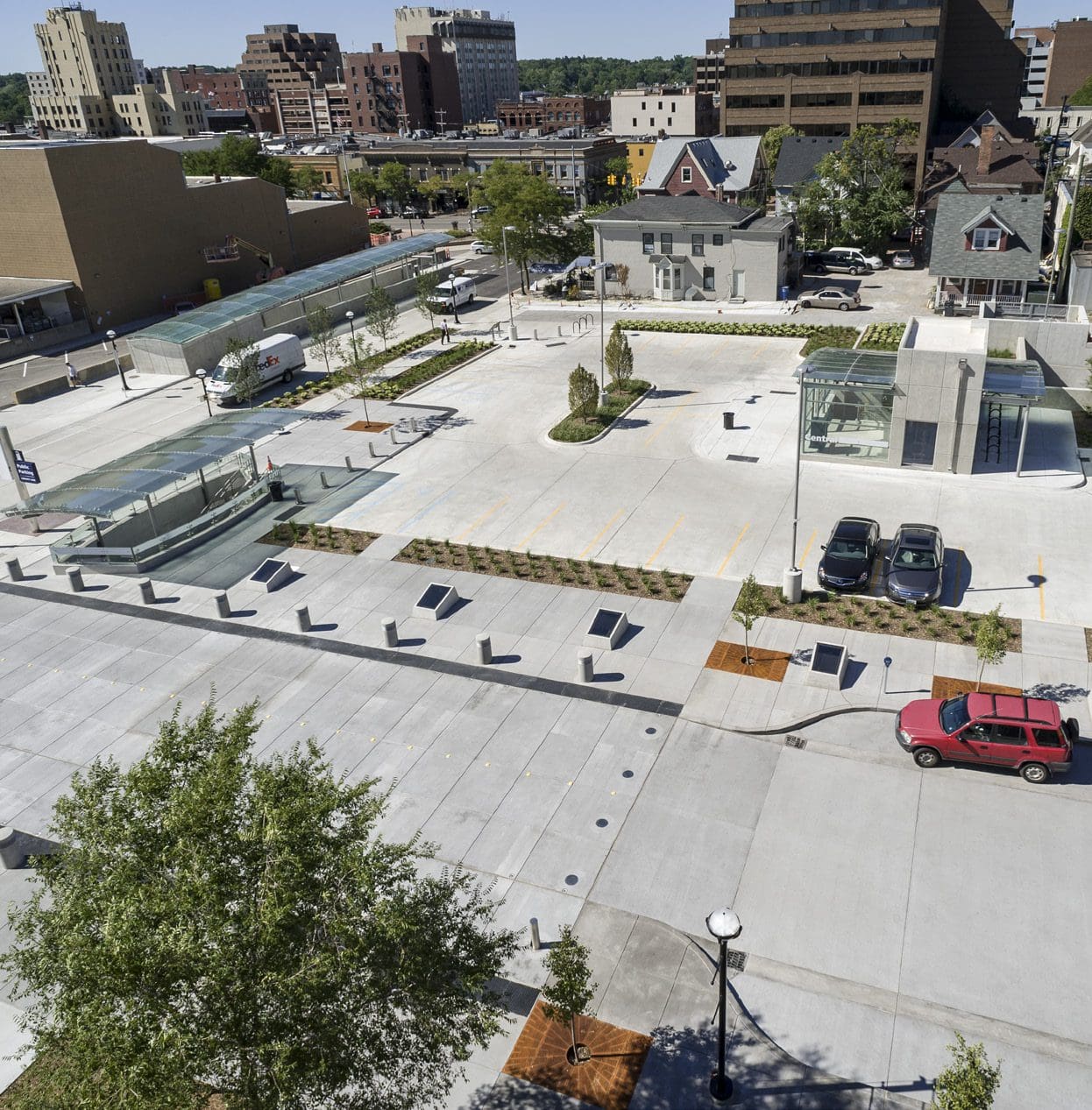The image depicts a top-down view of a light gray concrete parking lot with yellow lines demarcating parking spaces. Prominently in the middle of the lot, there is an oval divider filled with grass and featuring two trees growing from its center, as well as a silver-colored post. On the right side of the lot, two cars can be seen parked; one is dark gray and the other is black. In the bottom right corner, a red SUV is parked in front of a series of upward-angled squares that resemble solar panels. To the left of the parking area, there appears to be a gathering space or walkway with a tinted plastic covering. In the background, a street runs across the image, where a white FedEx cargo truck is visible. Further in the distance, there are various buildings, including tall brown ones and smaller structures, with a strip of blue sky and tree line visible beyond them. Additionally, some patches of grass with smaller bushes and decorations are distributed around the center divider, and there are stairs possibly leading down to a subway station or public transit area, indicating that this might be part of a downtown city square.